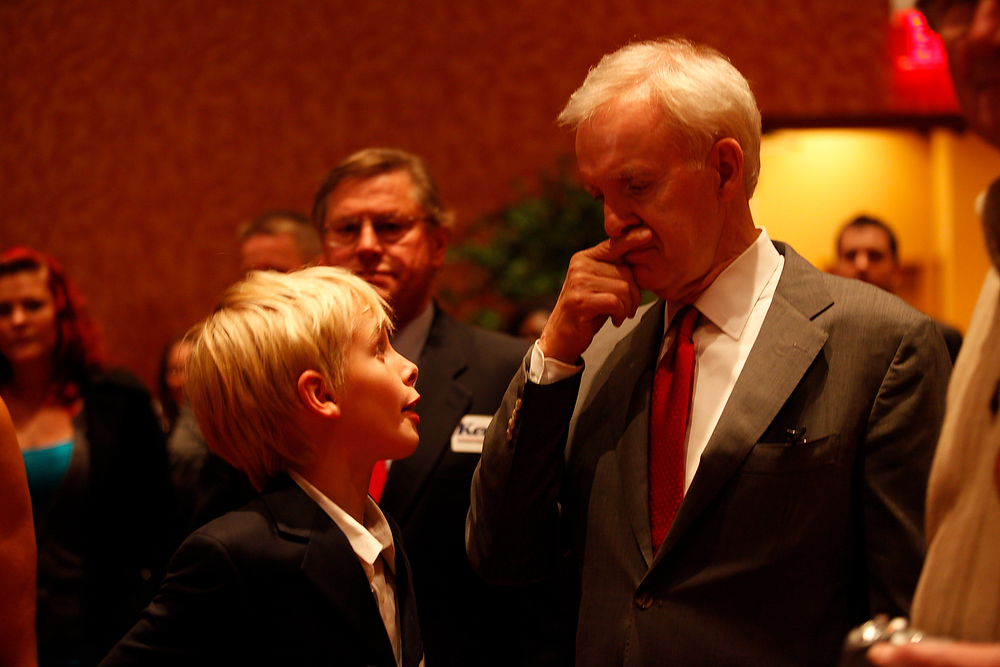The image captures a scene in a room with red wallpaper and various people in the background. At the center, a young blonde boy stands in front of an older man resembling the famous film director James Cameron. The boy, dressed in a black blazer over a white button-down shirt, looks incredulous and has very red lips. The older man, who might be Cameron, wears a gray blazer, a red tie, and a white shirt, and has white hair. He's intriguingly holding his index finger underneath his nose, perhaps pretending it's a mustache. The room's background is populated with two women and two men, with a green bush backed by the red wall and another man standing against a yellow wall near an exit sign. The setting, detailed with elements like a hotel ambiance, suggests the possibility of a fan or business convention.